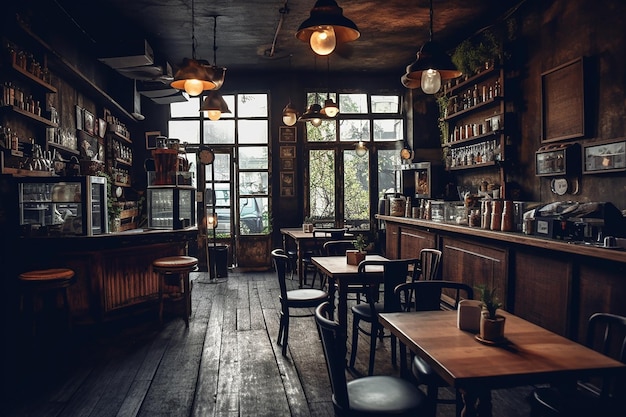The image captures the interior of a cozy coffee shop during daytime, although the shop itself remains dimly lit. In the background, windows on the center left and center right reveal a glimpse of the street outside, contributing to the ambient light. The left-hand side features a wooden bar adorned with two large glass display cabinets. Two bar stools are placed directly in front of the bar, inviting patrons to sit. Behind the bar, the back wall is lined with shelves holding various bottles and containers, reaching from the top of the wall to just below eye level. The wooden floor beneath is a warm, dark brown.

On the right side of the image, three tables are arranged in a line from the bottom right towards the center. Each table is equipped with wooden chairs and is quaintly decorated with small plants and containers in the middle. Behind these tables is another work surface, cluttered with various cups and containers, both on the surface and mounted on the wall above.

The ceiling boasts an array of hanging lights, each featuring a large lampshade and an orange-tinted bulb, casting a warm glow over the interior. The details and layout create a welcoming atmosphere perfect for relaxation.